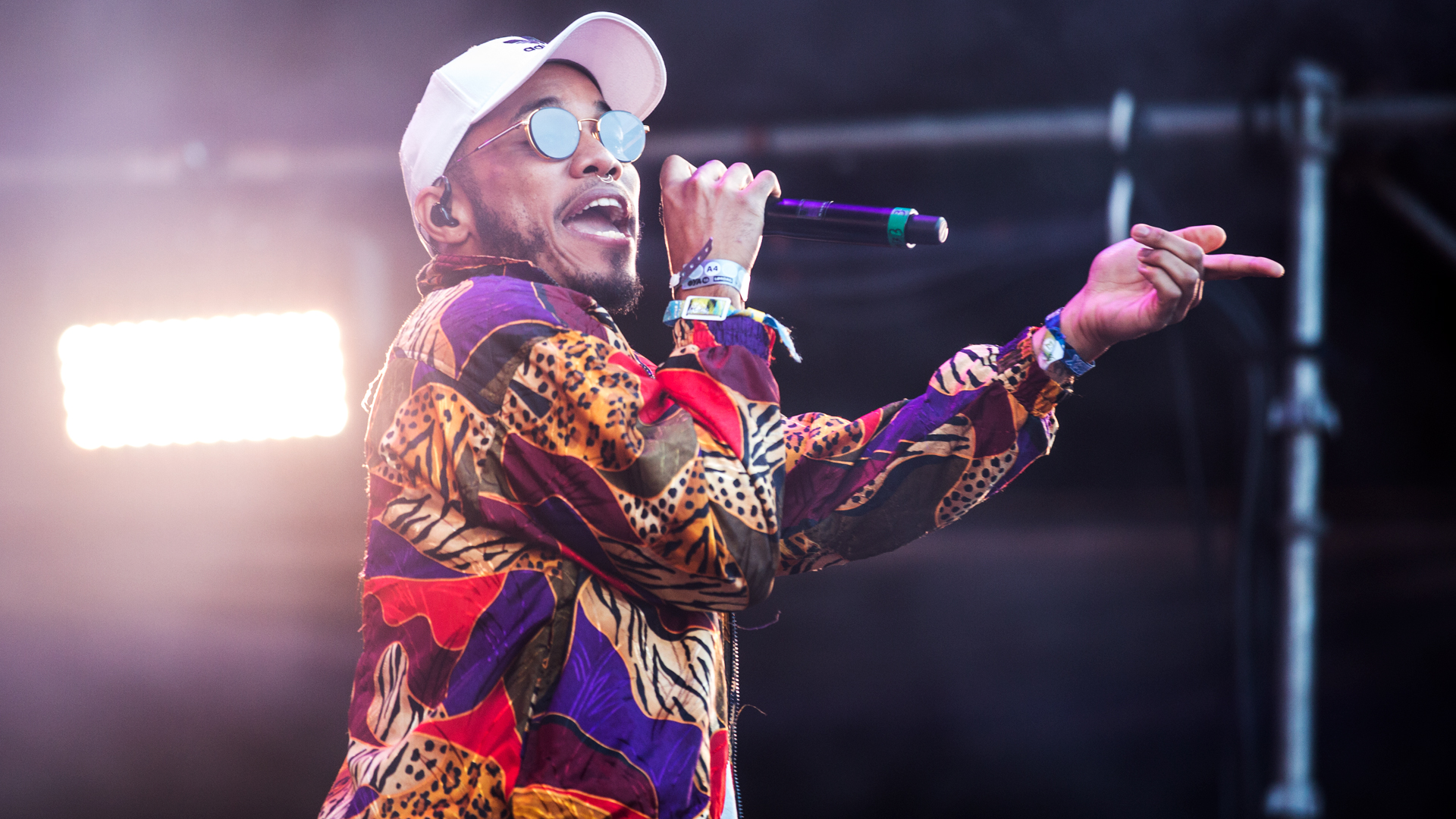The image captures a dynamic moment of a lively musician, a Black man with a light skin complexion, performing on stage. He is positioned in the center of the photograph, slightly turned sideways to the right whilst his head faces more towards the front. His mouth is open mid-performance, revealing his clean, white upper and lower teeth and his tongue, suggesting he's either singing or making an announcement. 

He is wearing a white ball cap and round sunglasses, with an earpiece discreetly fitted in his ear. In his right hand, he holds a distinctive purple microphone, and his left arm extends outward with his finger pointed, possibly engaging with the audience or indicating something of interest. His black goatee is framed by long sideburns, adding to his charismatic appearance.

His jacket is a visually striking piece, composed of a patchwork of vibrant colors and animal prints, including leopard and tiger stripes, alongside solid hues of purple, magenta, burgundy, and red. A bracelet, indicative of festival admission wristbands, adorns his wrist, hinting at the nature of the event.

The backdrop features the structural bars of the stage and a large spotlight on the left side of the image, blurred but prominent, contributing to the overall atmosphere. The stage setting, with its metallic structures and lighting, suggests that the scene could be an outdoor festival or an indoor arena concert, though it remains ambiguous whether it is day or night.